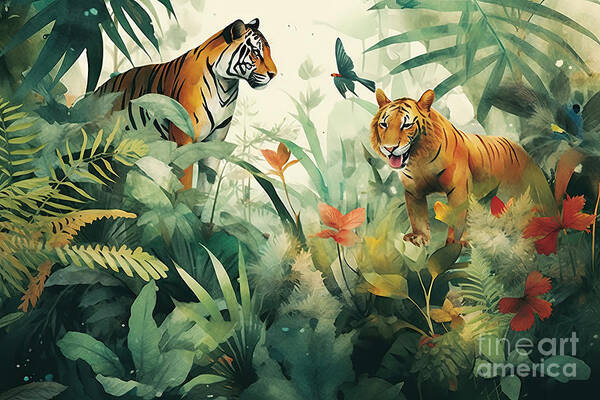This digital artwork, available from Fine Art America as indicated by its watermark on the bottom right-hand side in a mix of thin and bold fonts, vividly encapsulates a dense jungle scene with two striking tigers as its focal point. The tiger on the left, characterized by blank white eyes, gazes intently towards the tiger on the right. This right-side tiger, featuring pitch dark eyes, directly confronts the viewer with its mouth agape and tongue hanging out, providing a dynamic sense of panting. This contrast enhances the dramatic tension in the scene. Both tigers are adorned with classic orange and black stripes; the one on the right exhibits a more pronounced white facial pattern compared to its counterpart. The composition includes lush plant life with myriad green leaves and vibrant red flowers, creating an overwhelmingly green backdrop peppered with color. Amidst this jungle, a teal-colored bird with a striking red head soars, positioned closer to the tiger on the right. Despite the dense foliage, a soft fog veils the deeper jungle, adding a layer of mystique to the artwork.